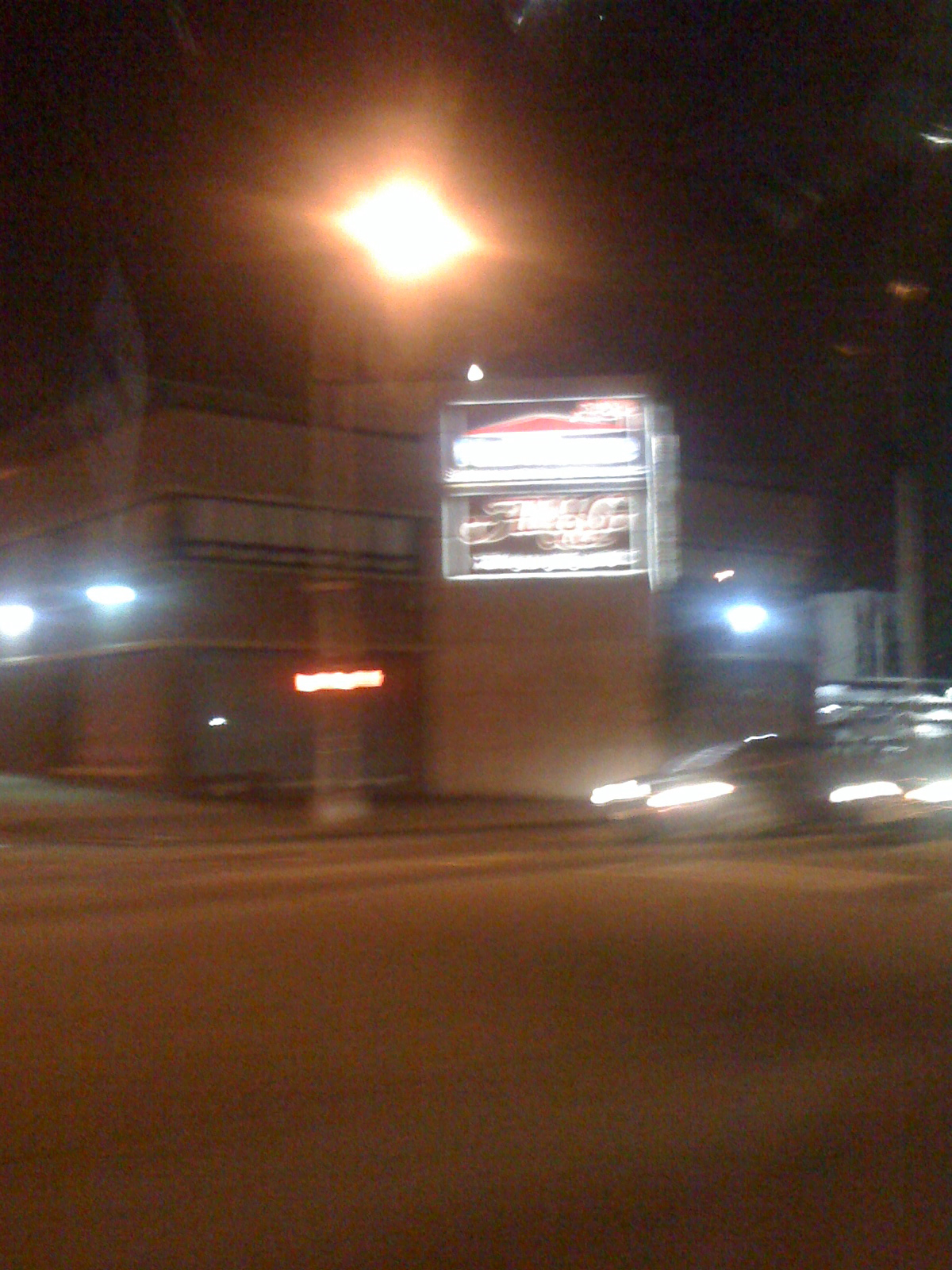This night-time photograph captures a scene drenched in a bronze-brown hue. The image, taken either out of focus or at high speed, is entirely blurred, giving it an abstract, painterly quality. In the background stands a building, its details obscured, but its presence dominating the frame. A massive spotlight in front of the building shines directly towards the camera, creating a powerful flare that obscures much of the scene beneath it. Below this intense light sits an illegible sign, adding to the enigmatic atmosphere. On the street in front of the building, two cars are in motion, their headlights streaking through the image and leaving only traces of light behind. The overall effect is a surreal, almost cinematic representation of a nocturnal urban landscape.